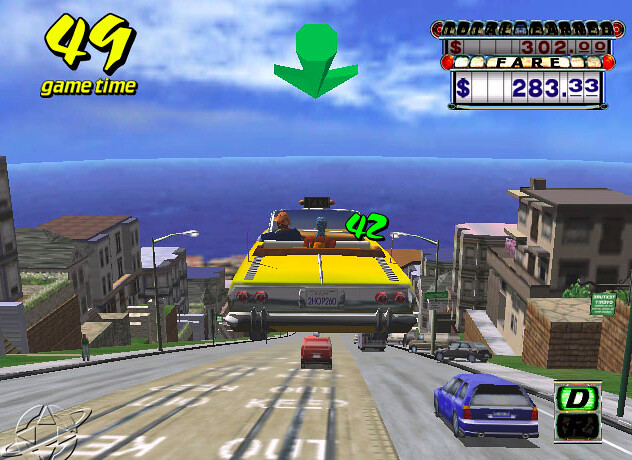In this screenshot from a video game, the top left corner displays "49 game time." The main focus is a California license plate affixed to a 1960s-style convertible, which resembles a taxi. The taxi is captured mid-flight, about to land on a street in what appears to be a quaint beach town. The scene includes a stunning ocean view straight ahead beneath a vast blue sky. Although the game isn't explicitly identified, it bears a striking resemblance to "Crazy Taxi," a popular game from the past. In the top right corner, a fare meter shows an accumulating total of $283.33.